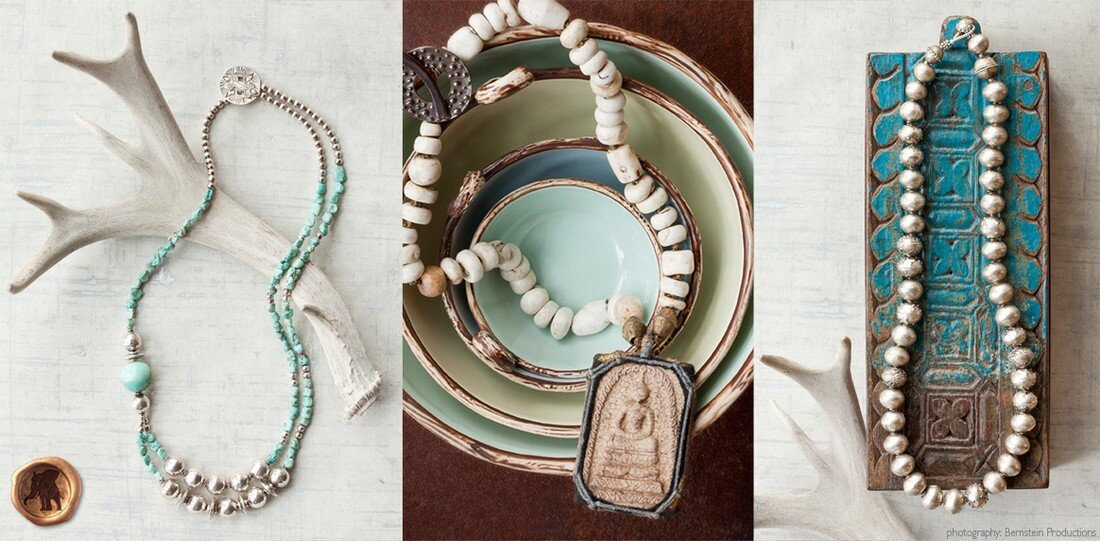This composite image features three distinct necklaces presented in a curated, artistic layout. On the far left, a necklace crafted from turquoise and silver beads is elegantly draped over a small, weathered branch set against a white background. This image includes a subtle gold emblem in the lower left-hand corner, possibly indicating a brand logo. The central image showcases a white stone necklace with a prominent Buddha pendant, resting atop a stack of bowls in varied hues of white, pale green, and turquoise blue, set against a warm brown backdrop. The final image on the right presents a necklace of pure silver beads reclining on a turquoise and dark brown decorative slate, with an additional weathered stick included in the composition against another white background.